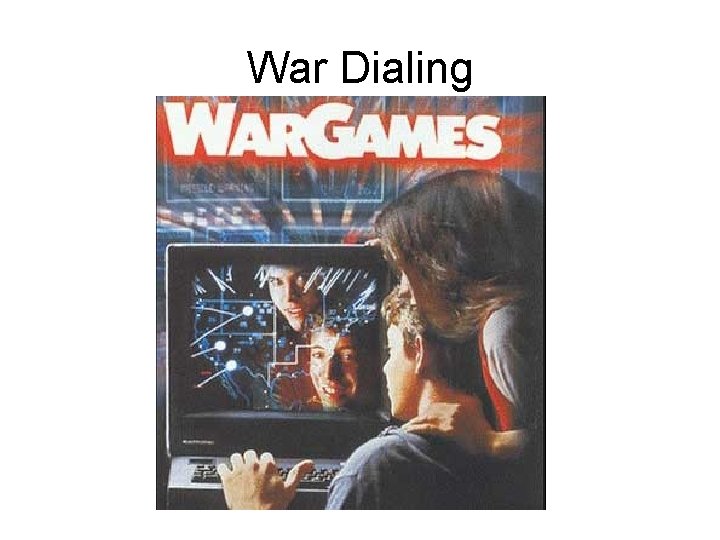This is a detailed advertisement for the classic 1980s movie "War Games." The title "War Games" is prominently displayed at the top in large, white, bold letters with a glowing red outline. In the image, a boy and a girl are positioned in front of an old computer, with the boy's hand poised on the keyboard. The girl, with long, dark brown hair, stands behind him, her hand resting on his shoulder as she looks intently at the screen. The screen itself shows a map of the United States with what appears to be missiles being dropped, adding a sense of dramatic tension. The reflections of the boy and girl, who have smiles on their faces, are visible on the computer screen, suggesting a sense of excitement and curiosity. The boy, identified as a young Matthew Broderick, appears engaged, believing he's playing a game, which is an essential plot point of the movie. The phrase "War Dialing" is written in black text above the main image. This visual is enhanced by multiple flashes of light around the characters, which heighten the sense of suspense and intrigue.